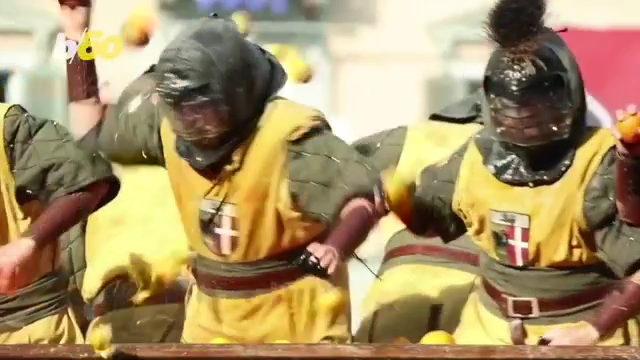In this captivating photograph, likely taken at a live-action role-playing event or a medieval sport reenactment, three participants are aligned side by side in the foreground. Each individual is clad in a distinctive ensemble, featuring a short-sleeve khaki green or camouflage green padded top. Over this, they wear a striking yellow tunic cinched at the waist by a green fabric belt, which is further secured by a leather belt. Prominently displayed in the center of each tunic is a heraldic badge, characterized by a white upper section bearing an inscription, a red flag with a white cross occupying the right side, and a dark image on the left.

Adding to their medieval flair, the participants sport leather cuffs extending from their wrists to elbows and padded helmets, each equipped with face protection. The person on the far right stands out with an additional plume adorning the top of their helmet or face covering. A wooden bar stretches horizontally across the bottom of the image, possibly part of the event setup. In the blurred top left quarter of the photo, several objects resembling balls are seen in mid-air, adding a dynamic element to the scene.

The background, slightly out of focus, reveals the backs of two more individuals dressed similarly in green and yellow tunics, immersing the viewer deeper into the event's atmosphere. The overall composition suggests an organized activity, rich with historical detail and vibrant in its presentation.